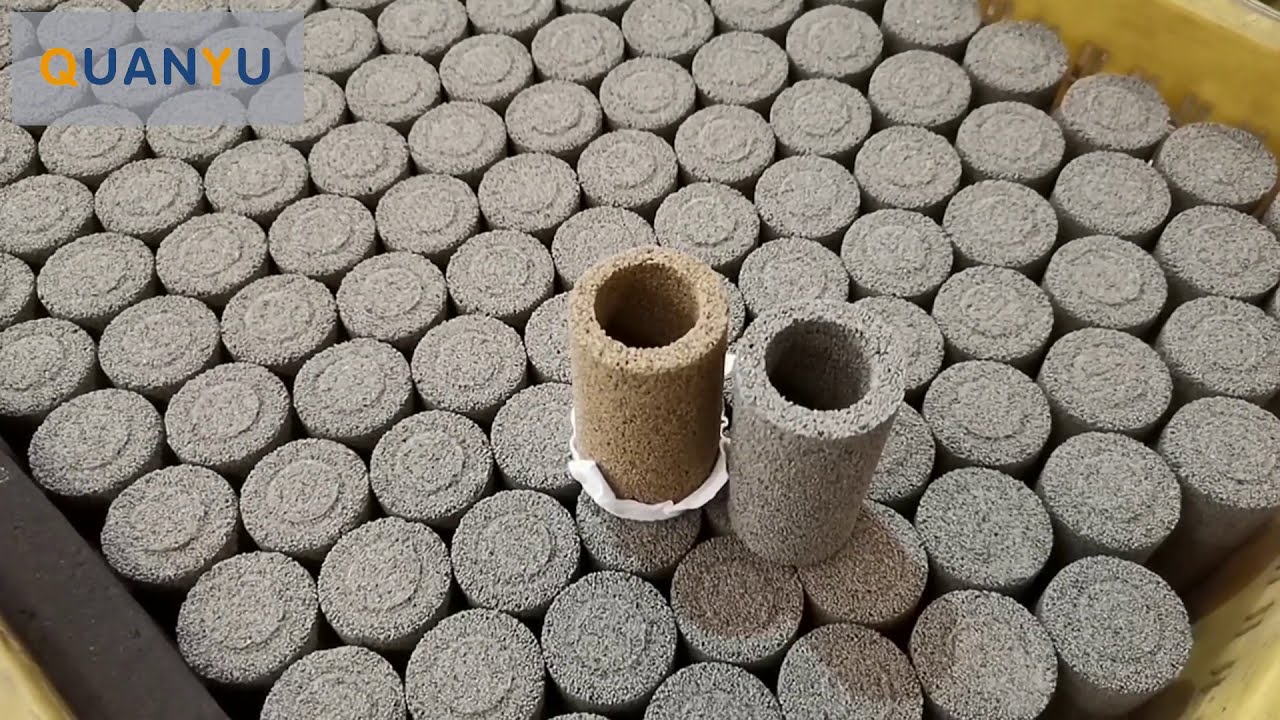The image portrays a slightly diagonal, wide rectangular aerial view of a yellow crate, seen partially in the top right, bottom right, and bottom left corners, with a gray strip near the bottom left edge. Inside the crate, numerous gray, cylindrical objects with a gritty, sandpaper-like texture are packed together, all having flat tops with slightly raised central portions. Among these, two distinct cylinders stand out in the middle right; one is gray and the other is tan, both open-ended resembling toilet paper rolls. Notably, in the top left corner of the image, the word "Kuan Yu" is displayed, with the letters ‘Q’ and ‘Y’ appearing in orange or gold, while the rest are in blue.